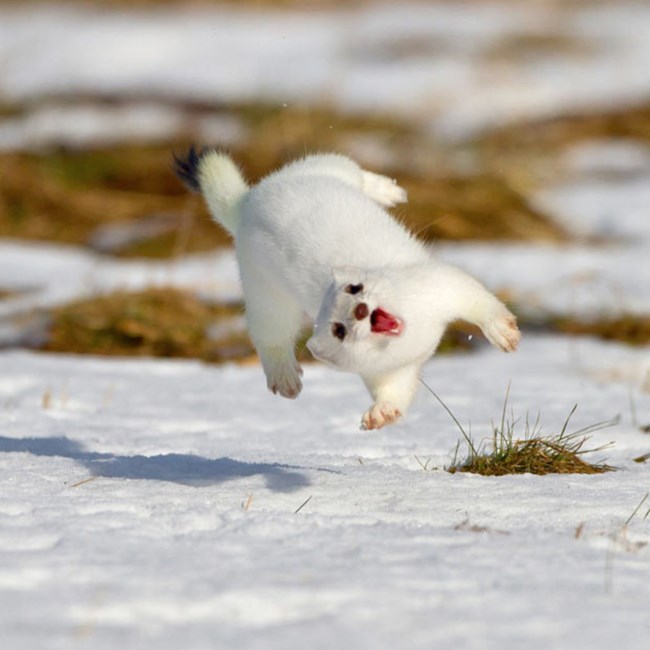In this detailed nature photograph, a small white ferret-like animal is captured in mid-air, leaping through a snowy landscape. The scene is set against a blurred background of a snow-covered field, with patches of dead grass or mulch subtly visible. The animal's thick, white fur suggests it is adapted to cold weather, likely for camouflage purposes. Its dark brown nose and very dark eyes contrast sharply against its white coat, while its small, rounded ears, fluffy tail, and extended paws give it an animated and lively appearance. The animal appears to be looking toward the camera with its mouth open, revealing little fangs and a surprisingly red interior, almost as if it's smiling or expressing surprise. Despite the wintry setting, the creature seems to be thoroughly enjoying itself, exuding a sense of joy and playfulness as it frolics in the snow.